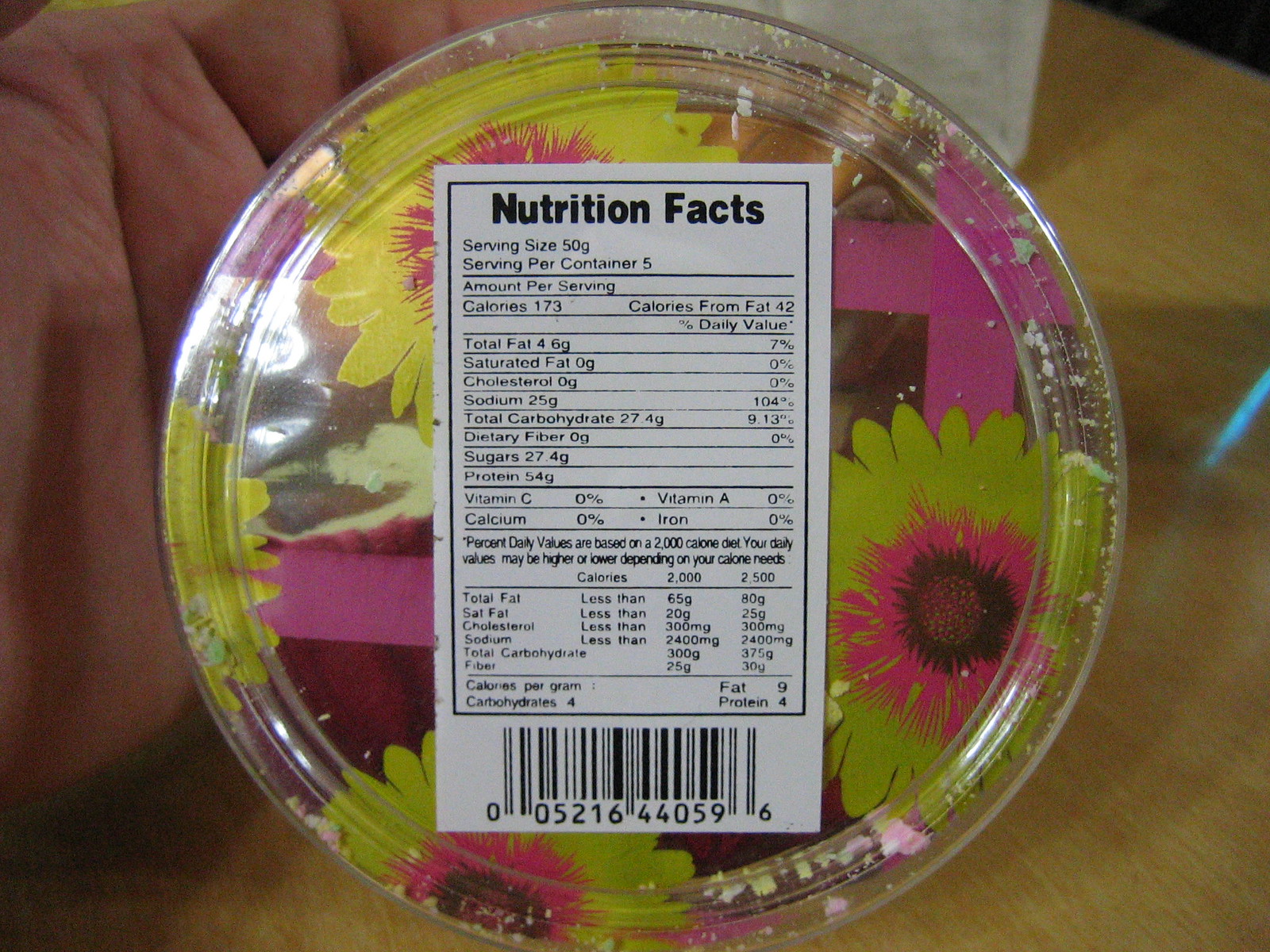The image features the back of a transparent plastic clamshell container prominently displaying a Nutrition Facts label at the bottom. The packaging design is adorned with large, vibrant yellow and pink flowers. The yellow blooms exhibit pink details surrounding their centers, which are tinged with brown. Additionally, there are pink stripes reminiscent of decorative tape integrated into the design. In the background, on the left side of the image, a hand holds up the container, presenting it to the viewers. To the right, the container rests on a table made of light-colored, finished wood, contributing to a warm and natural setting.